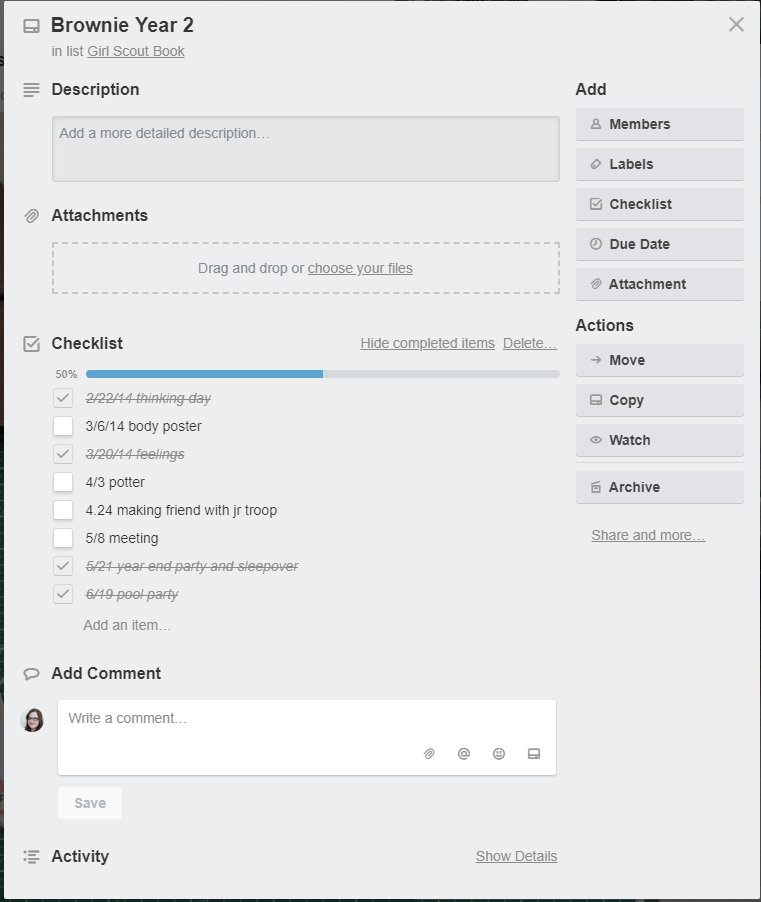This is a detailed and refined caption for the provided image:

The screenshot showcases a Girl Scouts tracking application tailored for the Brownie section, specifically for Brownie Year 2. The interface features a predominantly gray background and occupies a vertically rectangular space on the screen.

In the upper left corner, the bold black text "Brownie Year 2" distinctly marks the section of the Girl Scouts. Directly underneath, in gray and underlined, is the text "Enlist Girl Scout Book."

Below these headings, there are two designated areas: a description box followed by an attachment box. The main content area on the left side of the page prominently displays a checklist of activities, some of which are marked complete.

The checklist includes:
- **2-22-14 Thinking Day** (crossed out, with a checkmark in the box)
- **3-6-14 Body Poster**
- **3-20-14 Feelings** (crossed out, with a checkmark in the box)
- **4-3 Potter**
- **4-24 Making Friend with Junior Troop**
- **5-8 Meeting**
- **5-21 Year End Party and Sleepover** (crossed out, with a checkmark in the box)
- **6-19 Pool Party** (crossed out, with a checkmark in the box)

At the bottom of the page, there is an area designated for adding comments, providing a comprehensive and interactive tracking system for Girl Scout Brownie activities.